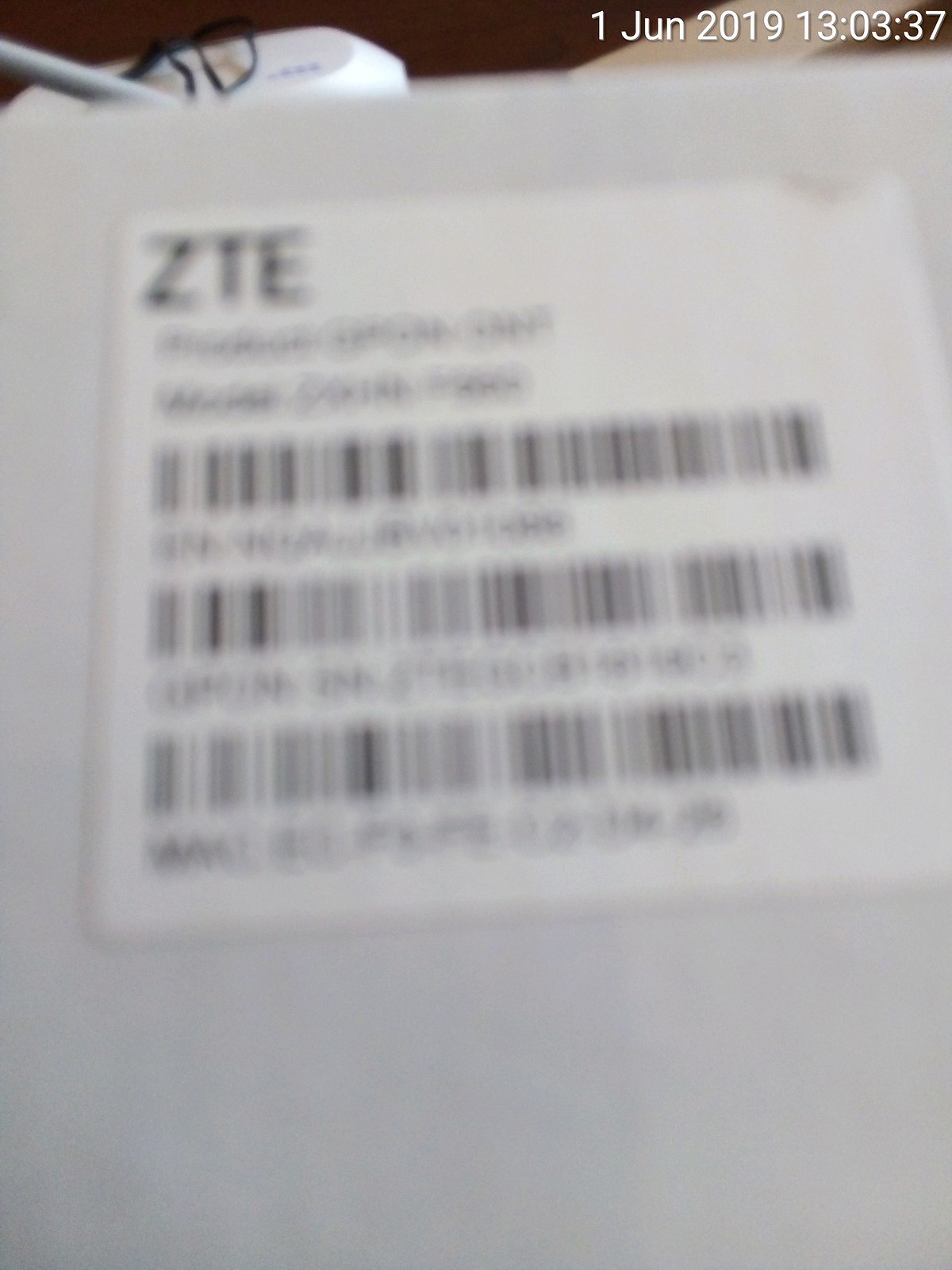The image is a close-up photograph of a white or light gray surface, possibly a box or a table, with a white sticker prominently displayed. The sticker features the letters "ZTE" at the top, and three distinct barcodes lined up from top to bottom. Below each barcode are some numbers or letters that are blurred and unreadable. In the upper right corner of the image, a digital timestamp reads "1 June 2019, 13:03:37." The top background of the image includes a mix of unclear objects, which might be a grayish cord, a piece of wood, a metal bar, and possibly a pair of glasses.